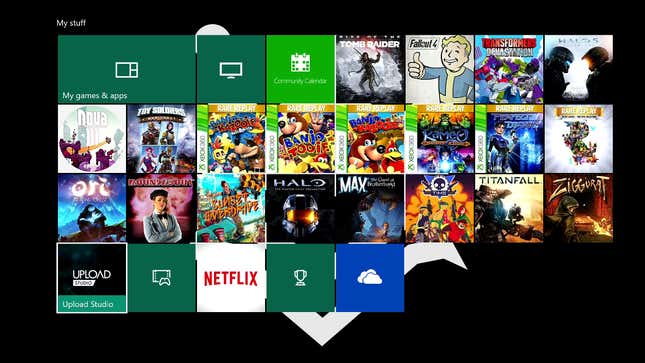This screenshot captures a page displaying a grid of various apps and games. The grid comprises four rows and eight columns of square-shaped icons, except for the top-left icon, which occupies two squares. The central theme is a mix of application icons and game covers. Dominated by green rectangles and squares with some displaying specific game covers, this layout offers a clear organization of media content.

On the top row, from left to right, we see a prominent "Community Calendar" occupying two squares, followed by "Tomb Raider," "Fallout 4," a "Transformers" game, and "Halo 5." Moving down the rows, additional entries include "Nova," "Dyad," "Toy Soldiers," and different iterations of the "Banjo-Kazooie" series, with "Banjo and Kazooie" featuring twice. At the very bottom, the "Netflix" app is also evident, rounding out the collection with a popular streaming service.

Overall, the arrangement presents a well-organized interface with a diverse selection of digital media at the user's fingertips.